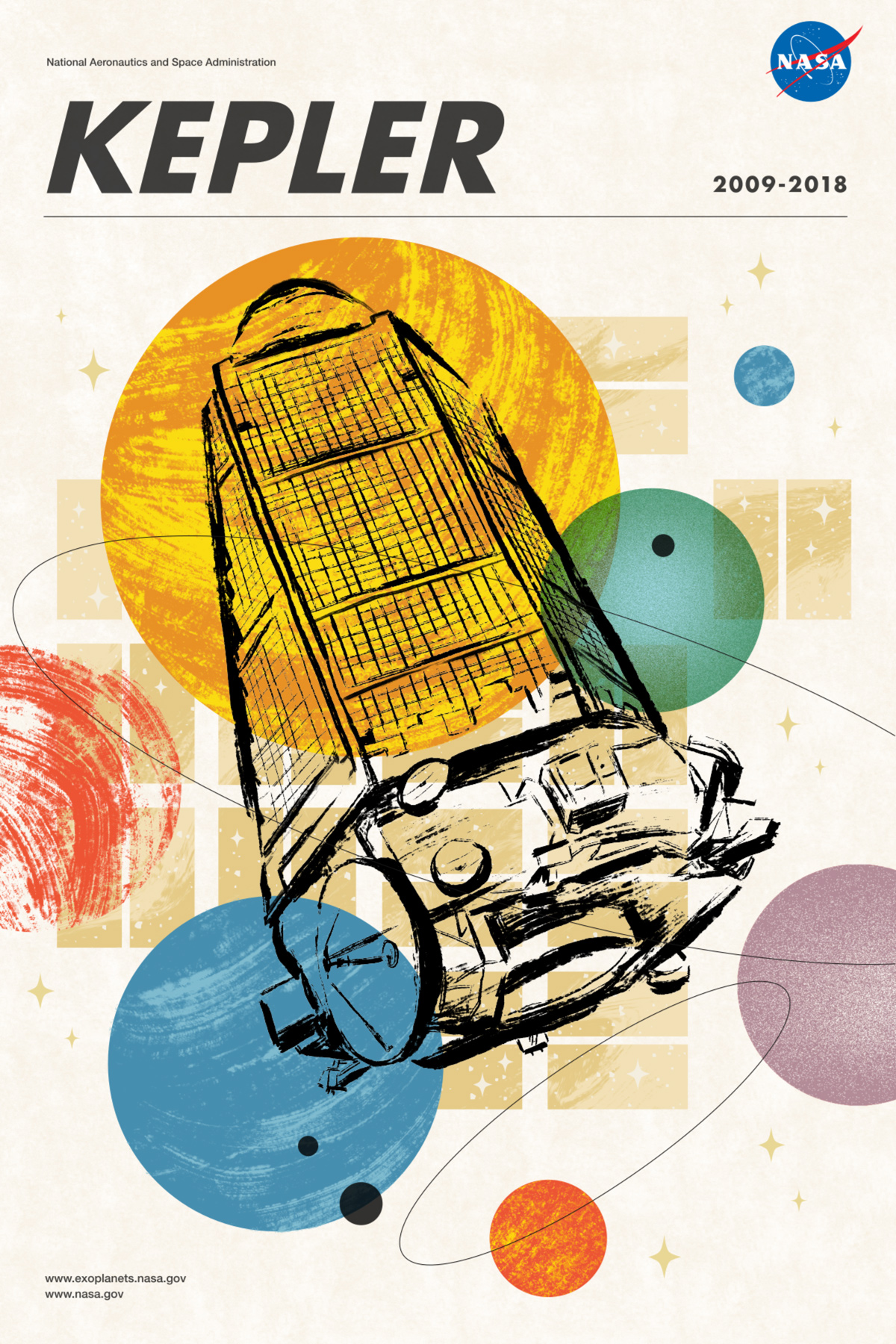The cover, reminiscent of a book or notebook from NASA, prominently features the bold title "Kepler" in large black letters on the top left. The iconic NASA logo is situated in the upper right corner, underneath which are the dates "2009 to 2018." The main artwork captures attention with its assortment of colorful spheres symbolizing various planets, set against a dynamic background. Overlaying this celestial scene is a detailed, hand-drawn depiction of a spacecraft, lending an animated and fresh feel to the illustration. At the bottom left, small text, presumably a web address for NASA, adds a final touch. Additionally, very small and hard-to-read black text spelling out "National Aeronautics and Space Administration" appears somewhere on the cover, tying the whole design together.